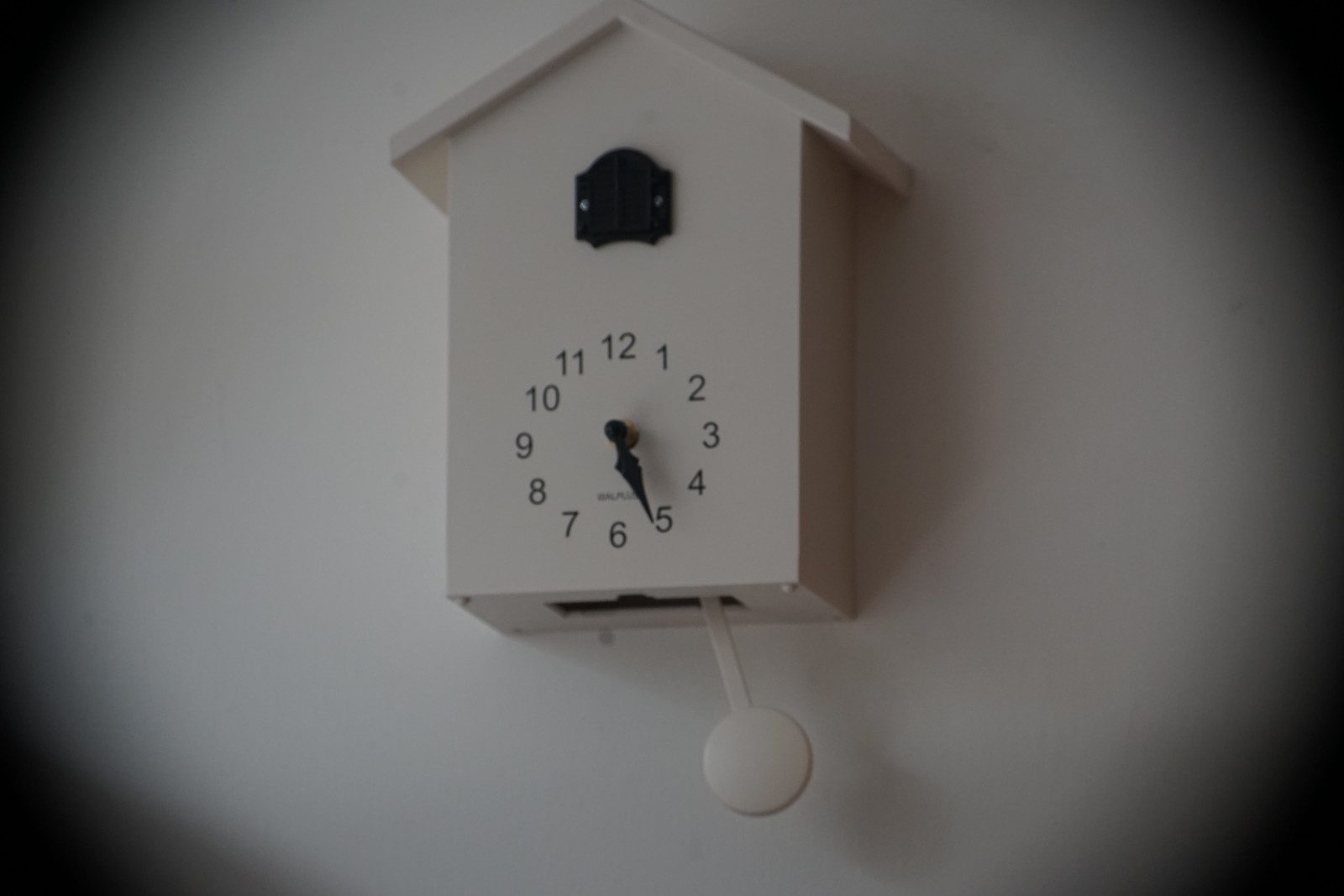The image showcases a charming, modern cuckoo clock with a sleek design that strays from traditional styles. The clock is predominantly white, which gives it a clean and contemporary look. A striking black door sits prominently in the center, from which a black cuckoo bird emerges. This contrast of black against white enhances the noticeable features of the clock. The clock face is adorned with black hands and numbers, further emphasizing the design contrast. Additionally, there is a pendulum-like bell at the bottom that appears to be swinging, a characteristic feature of traditional cuckoo clocks. The clock is mounted on a white wall, maintaining a minimalist aesthetic and drawing full attention to the clock itself.